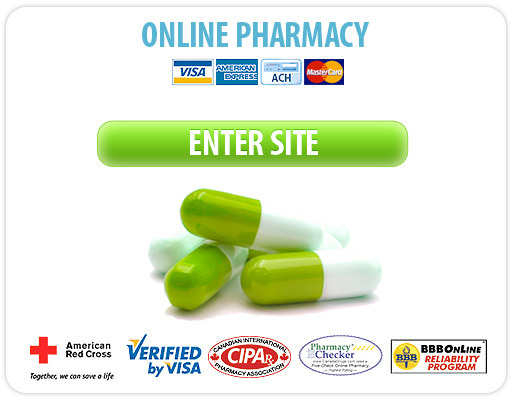The image depicts an online pharmacy webpage with a clean, white background. At the top, the page is labeled "Online Pharmacy" in light blue lettering. Below this heading are icons for several payment methods, including Visa (blue top, gold bottom, white middle with 'Visa' written over it), American Express (blue and white), ACH, and MasterCard (red and orange circles overlapping).

In the central part of the image, there's a prominent green button reading "Enter Site" in white letters. Scattered around the central button are three large green and white capsule pills. 

Near the bottom of the image, several logos and verifications are displayed. On the left is the American Red Cross symbol with the accompanying text, "Together we can save a life," written in black. Next to it, there's the "Verified by Visa" logo in blue. Further along, there are certification marks for the Canadian International Pharmacy Association (CIPA) and Pharmacy Checker, depicted in green and blue colors. Finally, on the right, there's the BBB Online Reliability Program mark, showing "BBB Online" in black lettering with red text for "Reliability Program" and a yellow circle featuring "BBB" in black letters.